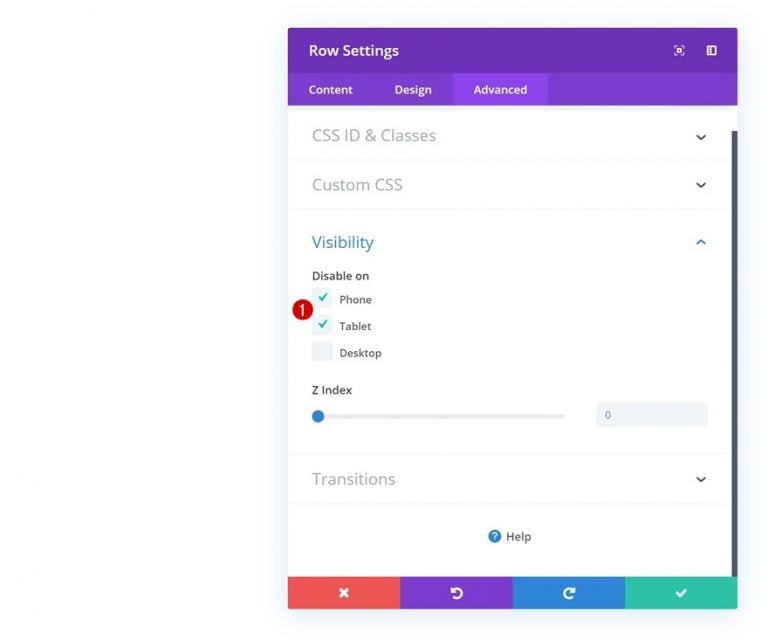Screenshot of a "Row Settings" Window

This detailed screenshot captures the "Row Settings" window with the following characteristics: 

- **Header:** The top section, including the header, is purple and prominently displays the title "Row Settings."
- **Tabs:** Just beneath the header are three tabs labeled "Content," "Design," and "Advanced."
- **Body:** The main body of the window has a white background and is divided into different sections:
  - **CSS ID and Classes:** The first section is dedicated to CSS ID and classes, with an accompanying down arrow on the far right.
  - **Custom CSS:** The next section is labeled "Custom CSS," also with a down arrow on the far right.
  - **Visibility:** This section stands out with its green text and includes options for disabling visibility on specific devices:
    - **Disable On:** Labels appear below "Visibility," presenting three checkbox options:
      - **Phone:** Checked with a green checkmark, accompanied by a small red circle with the number "1" to the left.
      - **Tablet:** Checked similarly with a green checkmark and a red circle with the number "1."
      - **Desktop:** Unchecked.
  - **Z Index:** A slider control labeled "Z Index" with a small bar indicating the value "0" is featured to the right.
  - **Transition:** The final section is "Transition," with another down arrow positioned on the far right.
  
- **Help Icon:** Positioned in the bottom middle of the screen is a help icon shaped like a question mark.
- **Footer:** The footer is multicolored:
  - **Icons on the Left:** An X icon with a red background.
  - **Middle Icons:** A back arrow with a purple background.
  - **Right Icons:** A right arrow with a blue background and a checkmark with a green background.

This image represents a concise yet comprehensive overview of each element and setting within the "Row Settings" window in a user interface.